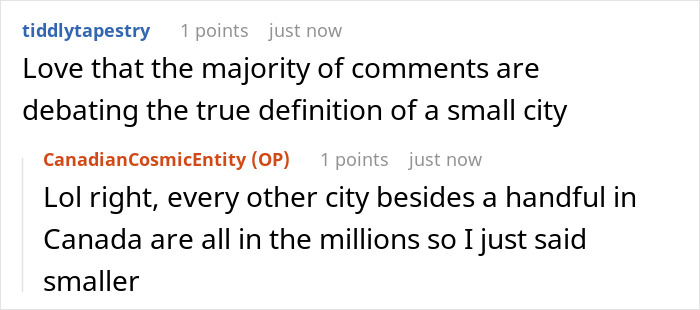This image is a screenshot taken from a forum-like website, capturing a conversation between two users. The usernames are color-coded differently from the text of their responses for clarity. 

The first comment is from "TiddlyTapestry," displayed in a blue font. The user has one point, and their message was posted just moments ago. TiddlyTapestry remarks, "Love that the majority of comments are debating the true definition of a small city."

The second comment is a response from "Canadian Cosmic Entity," the original poster of the thread. This username also shows one point and indicates that the reply was made only a short time after the initial post. Canadian Cosmic Entity responds with, "LOL, right? Laugh out loud. Every other city besides a handful in Canada are all in the millions, so I just said smaller."

The responses feature a noticeably larger font compared to the smaller, more subdued font used for the usernames, points, and post times. This screenshot is bordered by a thin black or gray outline, adding a subtle frame to the captured conversation.